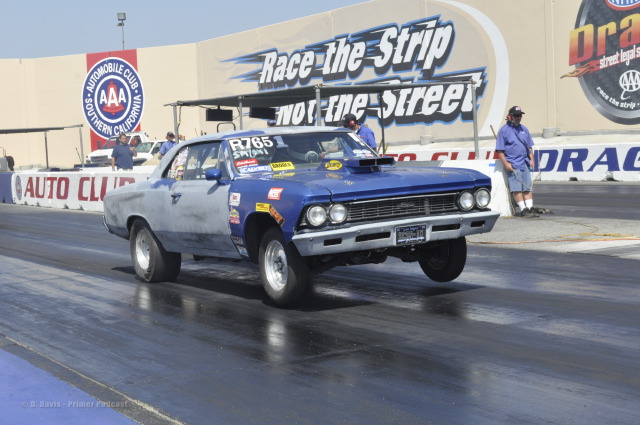The image captures a 1966 Chevrolet Chevelle drag racing car, characterized by its blue hood and front fenders, with primer gray doors, back, and roof. The car has just taken off on a black asphalt drag strip, with its front wheels lifted approximately three inches off the ground. The windshield features the number R6765, alongside various stickers. The background includes a white cement divider and several painted signs, including a blue circle reading "Automotive Club AAA Southern California," and another stating "Race the Strip, Not the Street." There are additional advertisements visible as well. Further back, there are maintenance workers wearing blue shirts and jean shorts, some with baseball caps, gathered under a covered area. The scene captures the dynamic and vibrant atmosphere of a drag race event.